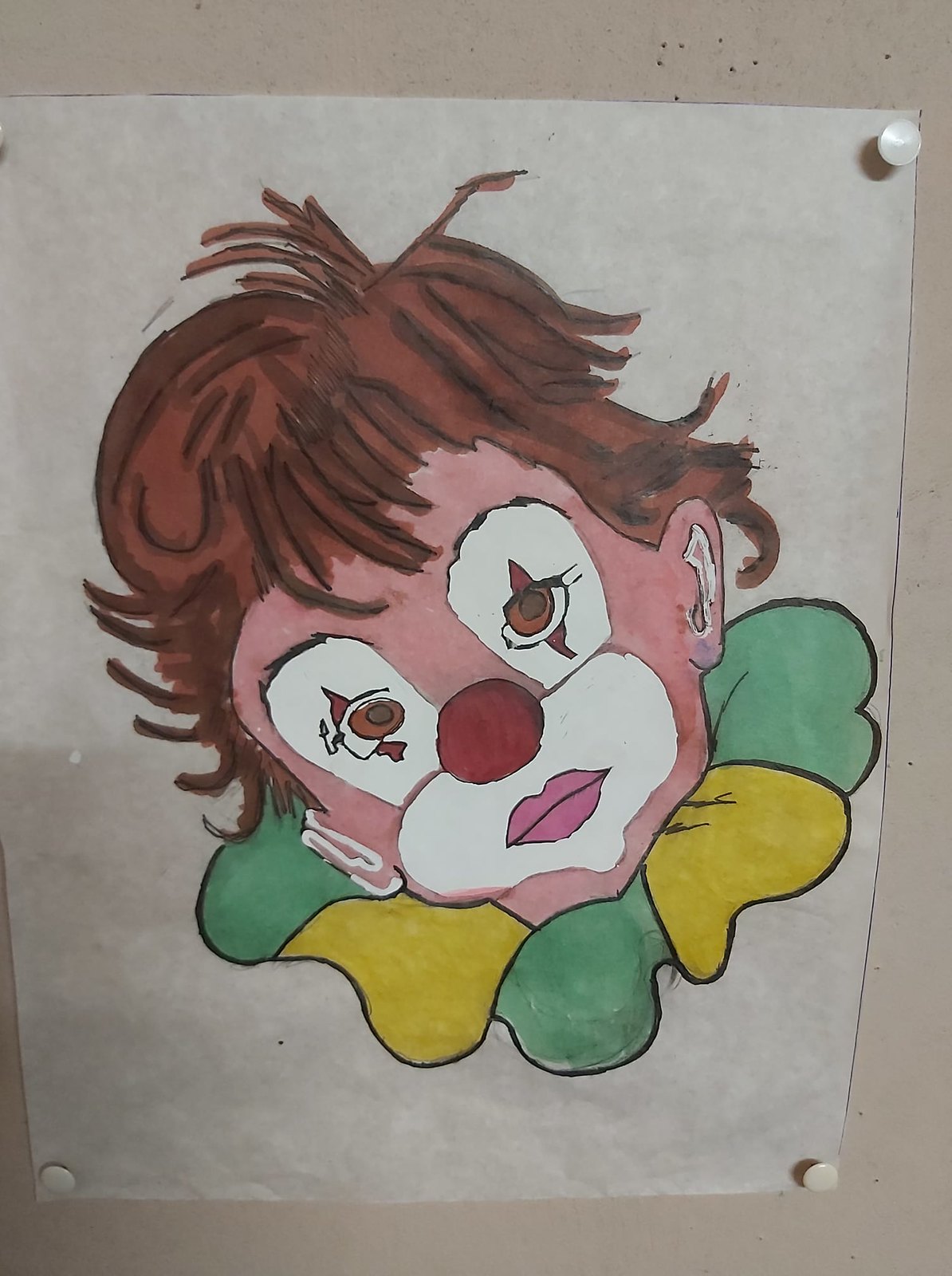The photograph captures a white piece of thin paper, pinned against a creamy grey wall with thumbtacks on three visible corners: a shiny silver one at the top right and two white ones at the bottom corners. The upper left corner is out of the frame. The paper features a watercolor or acrylic painting of a child-like clown face. The clown has disheveled brown hair outlined in black, a rosy pink face, white eye patches with brown pupils surrounded by diamond-shaped patterns, a large red nose, and pink lips. The mouth and chin are framed by a large white area. The clown's neck sports a ruffled collar with green and yellow sections accented by black outlines. Blue lines decorate the left and top edges of the paper, perhaps suggesting a border. The clown's expression is neutral, with no hint of a smile.